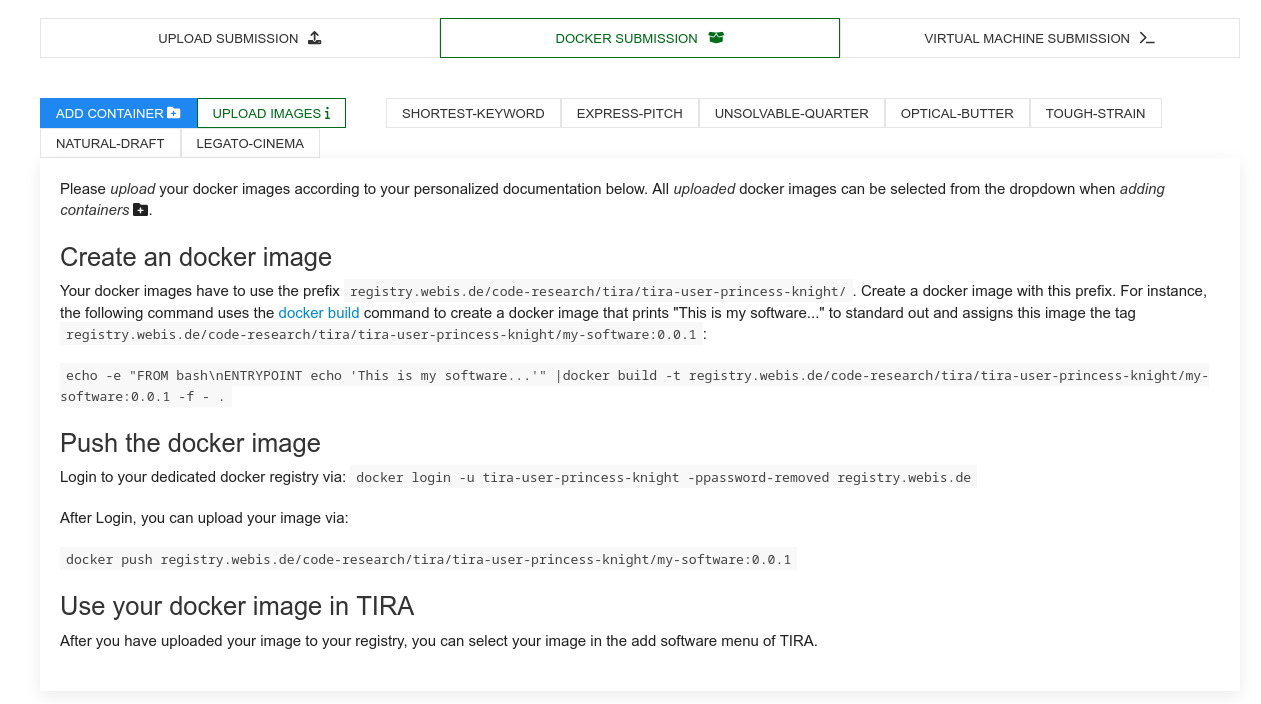This screenshot showcases an upload interface for a web platform or software. The top of the screen features three rectangular buttons labeled "Upload Submission," "Docker Submission," and "Virtual Machine Submission." The "Docker Submission" button is highlighted with a green border and green text. Below this, on the left side, there are two colored buttons. The first button, "Add Container," is blue with a folder icon. The second button, "Upload Images," is green. To the right of these, there are five rectangular buttons labeled "Shortest Keyword," "Express Pitch," "Unsolvable Quarter," "Optical Butter," and "Tough String." Additionally, below the "Add Container" button on the left, are two red buttons labeled "Natural Draft" and "Legato Cinema."